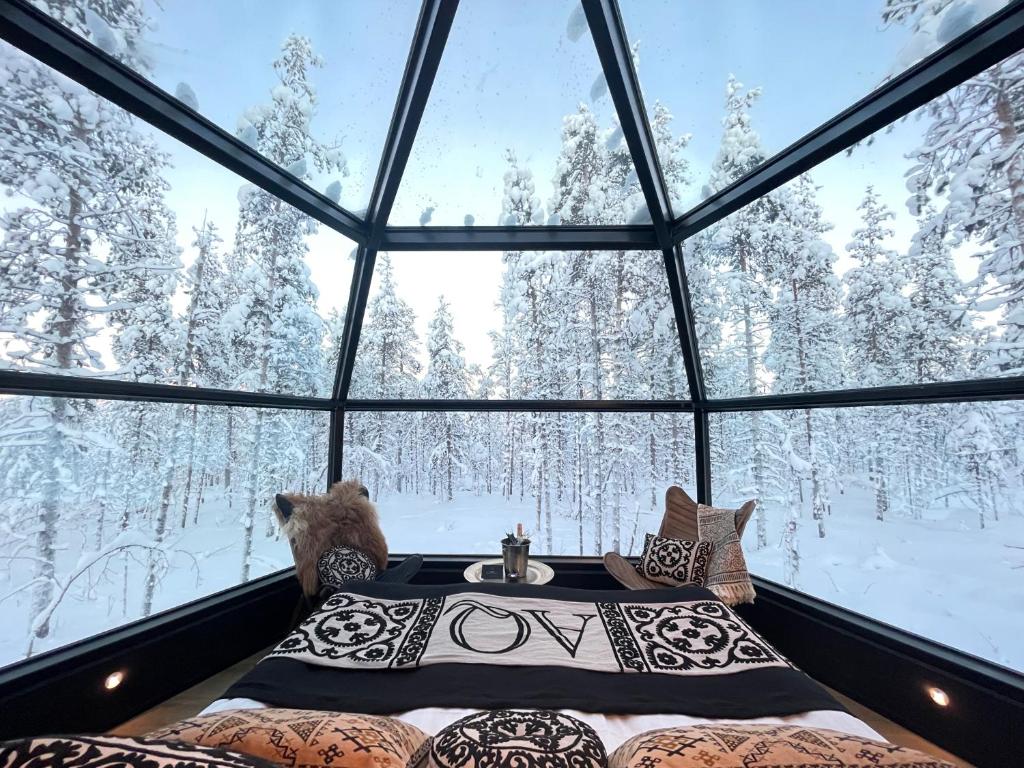This image is a color illustration, capturing an interior view from within a glass-walled room, shaped as a dome. The transparent walls allow a panoramic view of a serene, snow-covered forest, where every tree and the forest floor are blanketed in white. The sky is a light blue backdrop to the wintery scene outside.

Inside the room, there is a mattress or a futon laid out on the floor, with brown pillows. Draped across the end of the mattress is a large blanket with a black and cream design and the letters "AQ" prominently displayed. Adjacent to the foot of the bed, there are two chairs: one adorned with animal fur and the other with a blanket, each accompanied by black and white pillows. Between these chairs sits a round table that holds a metal bucket with champagne.

Space is available to walk around the bed, and the room is softly illuminated with lights around its base. The structure of the glass panels curves subtly towards the top, enhancing the feeling of being enclosed yet connected to the exquisite snowy landscape. The illustration presents a 3D, color-enhanced depiction of this cozy, modern sanctuary amidst a winter forest.